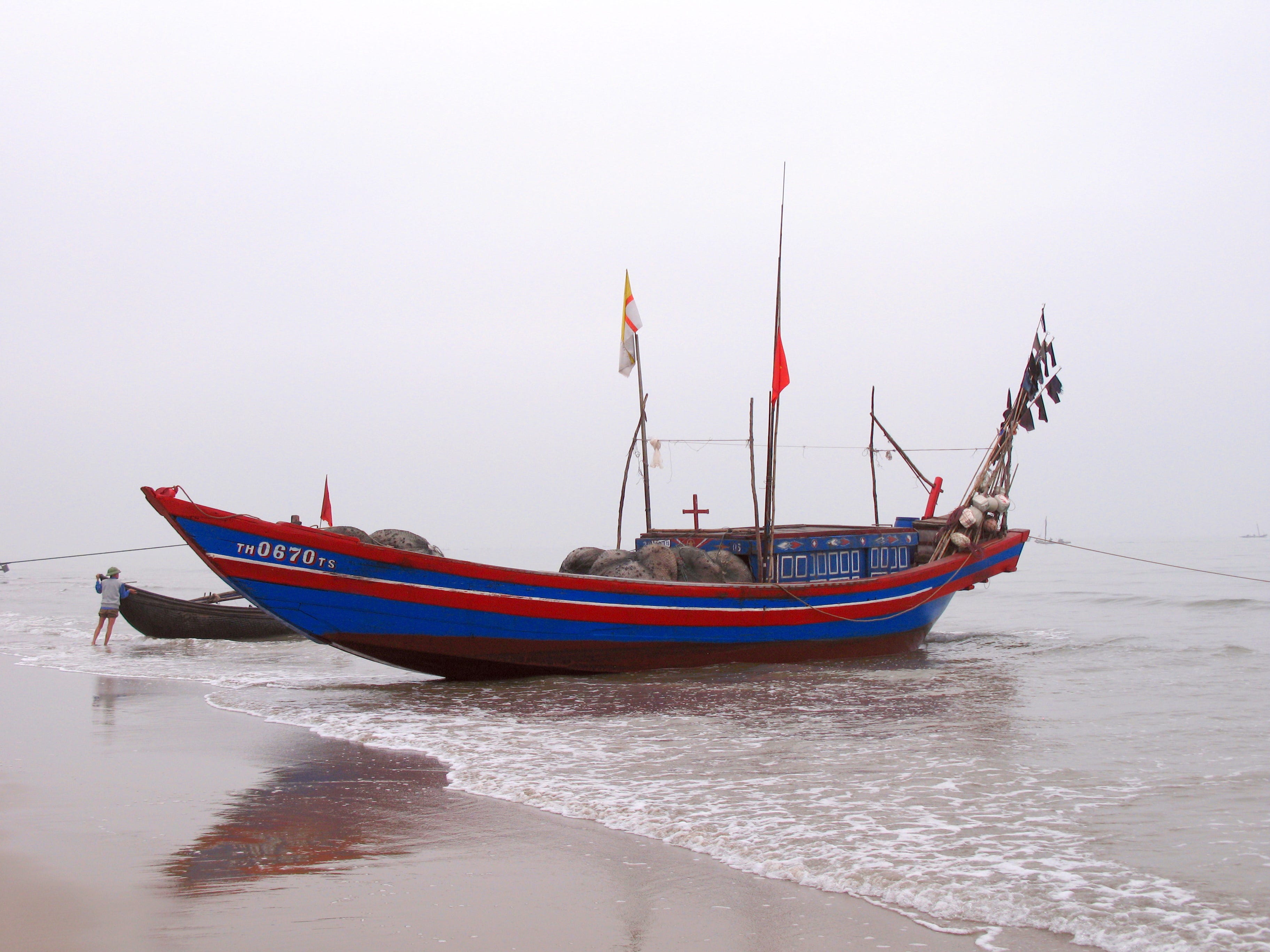This is an image of a small, brightly colored boat docked on a pale, faded sandy shore under a purpley-gray sky. The boat, centrally positioned, is predominantly blue with striking red trim and an additional red stripe. The distinct lettering "TH0670TS" is displayed on its side. Several flags adorn the boat, including a small red flag at the bow, a larger red flag in the middle, and a multicolored flag in white, orange, and yellow amongst other small pieces of material and sticks at the stern. A prominent red cross stands on a platform in the boat's center. The vessel, seemingly a fishing boat, contains rocks within or near it. The scene's backdrop includes an individual standing by an extremely small boat in the vast expanse of water with wet sand reflecting the diverse atmospheric hues.